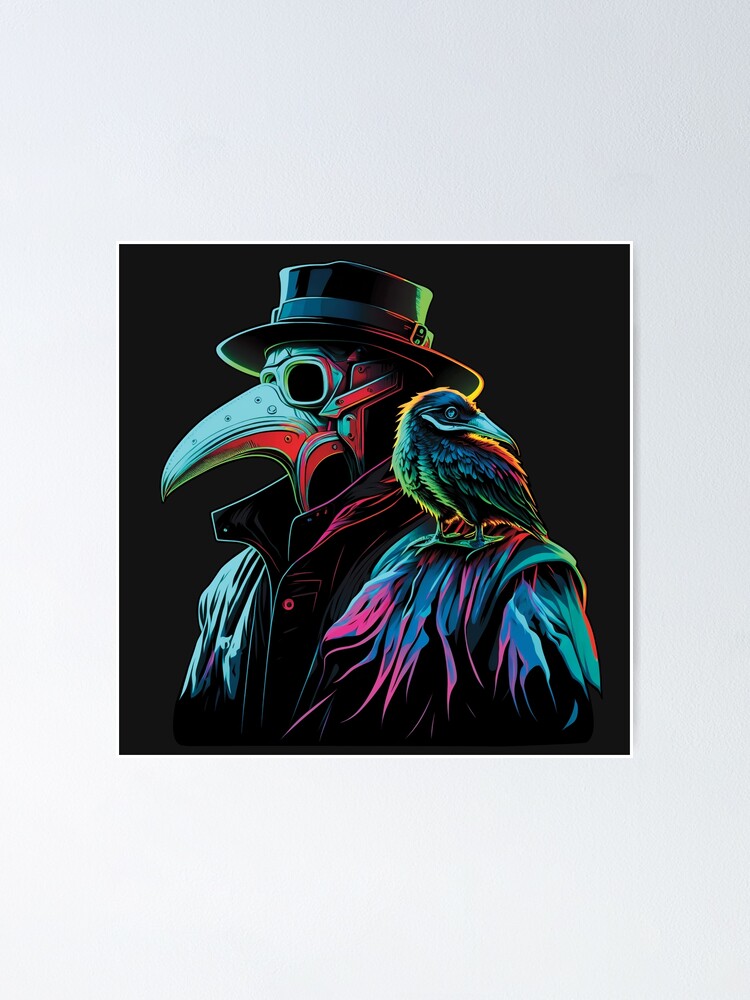The illustration depicts a vibrant and stylized figure set against a solid black background. The figure, reminiscent of a plague doctor, wears a round black hat with neon green, yellow, and red reflections. The character features a light blue mask with a long, pointy metal beak that has a red-orange glow at the tip. The dark jacket, accented with bright neon pink and blue highlights, has its collar turned up, and the entire composition of the figure exudes a glowing effect. On the character's shoulder sits a dark-colored bird with orange, yellow, green, and red highlights, adding to the illustration's vividness. Overall, the image is a striking contrast of dark and brilliantly luminous colors, making the figure and its companion stand out boldly against the black canvas.